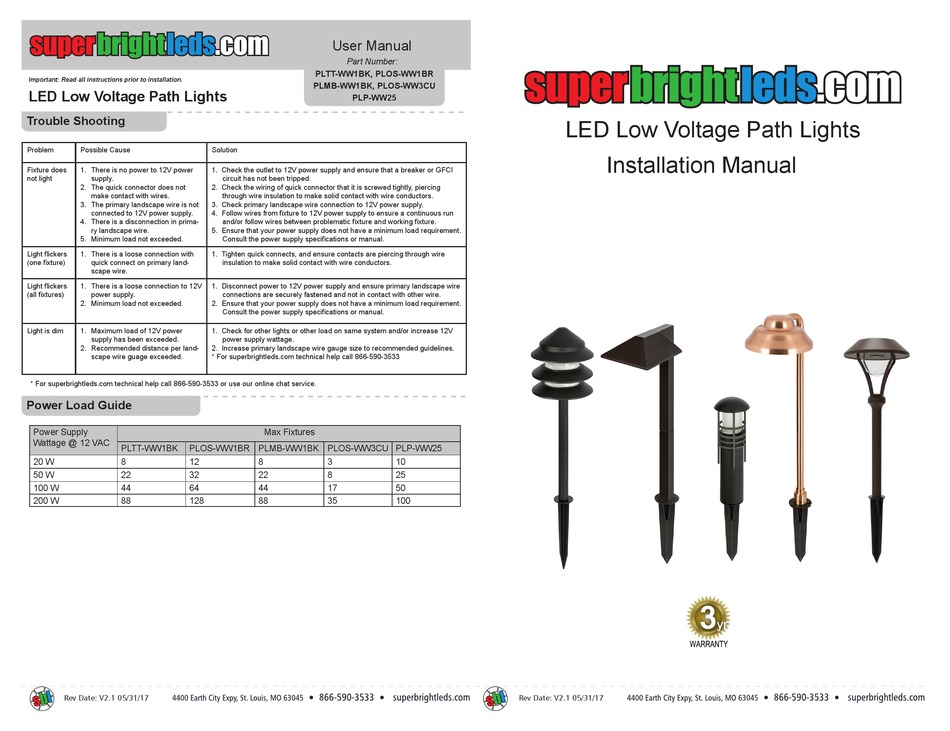This image depicts a webpage from an online retail store specializing in lighting products, specifically low voltage LED path lights. At the top of the page, the website's name is prominently displayed as "Super Bright LEDs" in vibrant red, green, and blue colors, while the rest of the text is in black and white. Below the header, a section titled "Troubleshooting" offers guidance to users experiencing issues with their lights. The troubleshooting box lists common problems, such as "Fixture does not light," "Light flickers (one fixture)," "Light flickers (all fixtures)," and "Light is dim."

On the left side of the page, there's another section labeled "Power Load Guide," likely providing information on how to properly power the lights. Adjacent to this, on the right side, the brand name "Super Bright LEDs" is reiterated, followed by a section titled "Low Voltage Path Lights Installation Manual." This section includes a series of images depicting various designs of low voltage path lights. There are five distinct designs showcased in the bottom right corner of the page, including a round, pagoda-like shape and a triangular one. The lights vary in color, with one having a brownish copper hue and the others being black. Each design features long poles meant to be installed into the ground, offering practical and aesthetically pleasing illumination options for pathways.